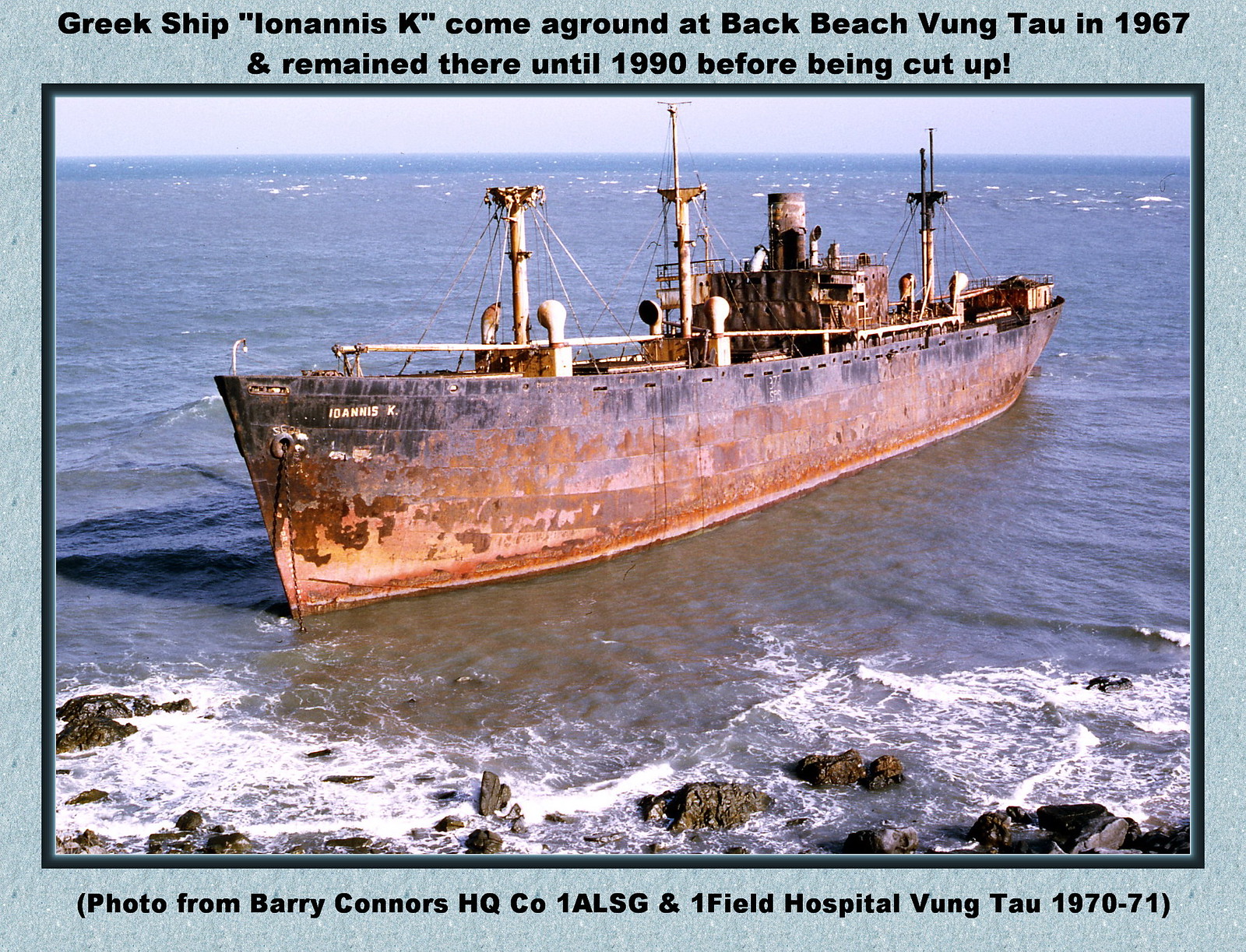This detailed photograph depicts the Greek ship "Ioannis K." marooned off the rocky shoreline at Back Beach, Vung Tau, Vietnam. The ship, displaying significant age with a rusted brown hull contrasted against dark blue side walls, has remnants suggesting it was already old when it grounded in 1967. It remained a poignant fixture until its dismantling in 1990. The surrounding sea presents a calm blue hue, reflecting a light blue sky. The scene, seen from a slightly elevated angle, shows the sun low in the sky, casting afternoon light on the vessel. This historical photo, bordered in dark and light blue, includes inscriptions detailing its origins: "Greek ship 'Ioannis K.' come aground at Back Beach, Vung Tau in 1967 and remained there until 1990 before being cut up." The credit at the bottom states, "Photo from Barry Connors HQ CO 1 LSG & 1 Field Hospital, Vung Tau 1970-71."